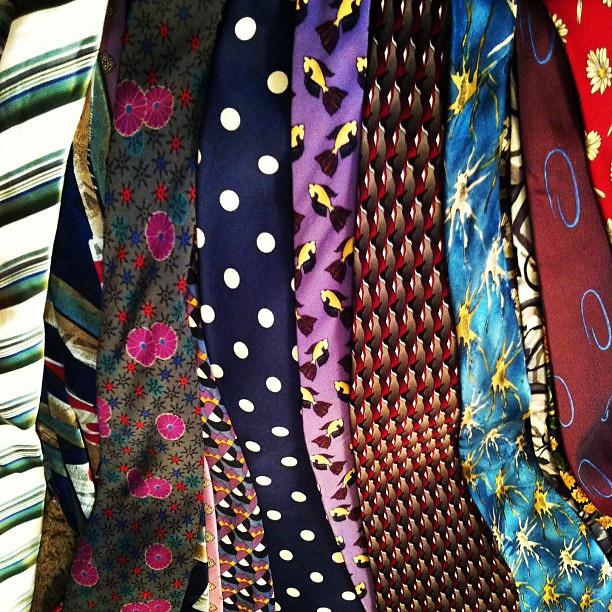This photo showcases a striking assortment of men's ties, arranged closely together, filling the entire frame with their vibrant patterns and textures. The collection features a diverse array of colors and designs, making it ideal for anyone looking to sell ties on platforms like Poshmark or Craigslist. Among the ties, there's a red one adorned with yellow flowers, another maroon tie displaying blue circles, and a blue tie featuring yellow and white fireworks or flowers. There's also a distinctive red and black tie reminiscent of motel carpet, a purple tie emblazoned with what looks like Oscar awards, and a blue tie with classic white polka dots. Additional ties include a grey one with red and orange accents that also evokes the feel of motel carpet, an unattractive grey tie with flowers, and a white tie with green, blue, and unappealing stripes. On the left side, a striped tie combines light tones with brown, blue, and green stripes, while a darker tie features pink flowers. There’s also a blue or purple tie with a whimsical fish pattern, and a light blue tie with splatter marks, each tie hanging down prominently from top to bottom. The overall impression is one of silky, fashionable fabrics, with prints ranging from paisley to geometric and animal designs, all vibrant and detailed, making this a compelling close-up that solely focuses on the rich fabric patterns.